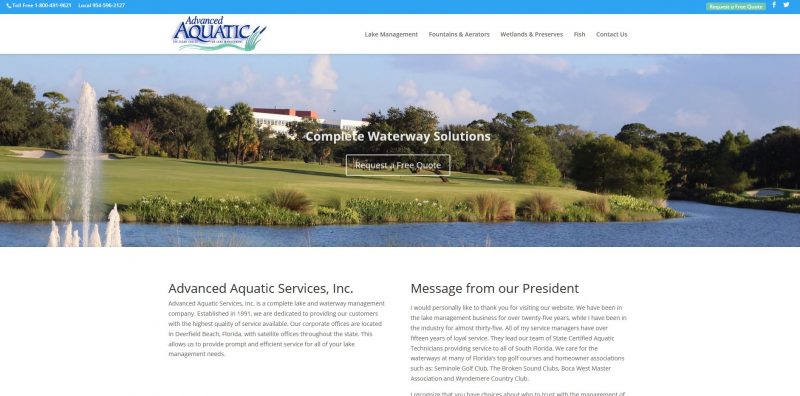Screenshot of a webpage featuring a serene aquatic theme. The top section is shaded in baby blue with somewhat illegible white text. At its center, there is an image resembling a generic phone, along with some text and two 1-800 numbers displayed. The upper right corner features text in teal green with white letters, next to recognizable Facebook and Twitter logos.

Below, on a white background spanning about a quarter of the page, bold dark blue text reads "Advanced Aquatic" with green text resembling aquatic weeds underneath. To the right, in black, are the services listed: "Lake Management, Fountains and Aerials, Wetlands and Preserves, Fish, Contact Us." A picturesque pond with lush green grass occupies the upper right, enhancing the backdrop.

Centrally, in white text, the slogan "Complete Waterway Solutions" is prominently displayed. Adjacent to this, a white text block reads "Request a Free Quote." Below, the company name "Advanced Aquatic Services Inc." appears in black, followed by additional unreadable text. On the right side, a section titled "Messages from our President" contains a passage of black text that is difficult to discern.